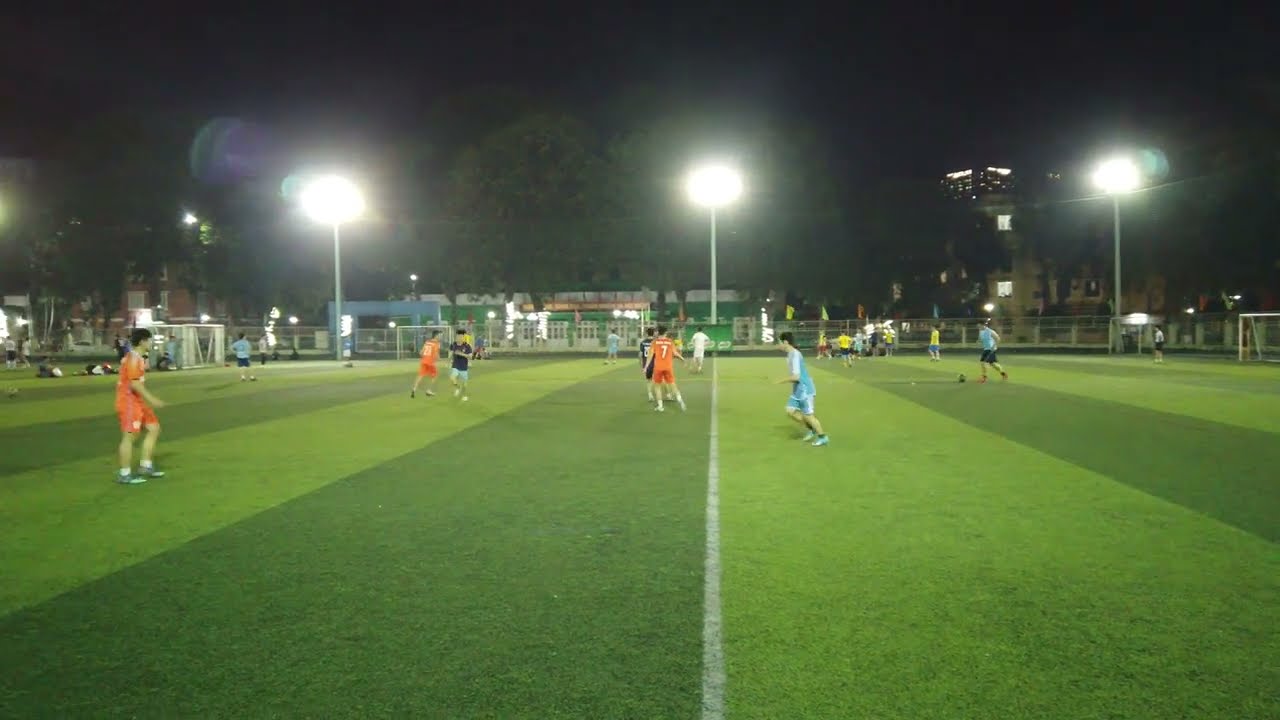The image captures a wide rectangular view of a nighttime soccer game on a field, consisting of alternating dark green and light green turf stripes extending towards the horizon. The field occupies the bottom half of the image, with soccer goals positioned at the middle right and middle left. The match depicts two teams of young men, identifiable by their distinct uniforms – one team in light blue and white, and the other in orange and white, with more players wearing orange jerseys. A white line is painted down the center of the field, and a ball is visible on the right side, being kicked by a player in a light blue uniform.

The game is illuminated by three bright floodlights, one centrally located and the others positioned on either side, set against a black night sky. The background reveals bleachers, tall lights, some trees, and a tall building with its lights on in the top right corner. Additionally, people can be seen in the bleachers, possibly wearing yellow. The surrounding scene, combined with the active players moving towards the center of the pitch, indicates an intense and dynamic moment of the soccer match.